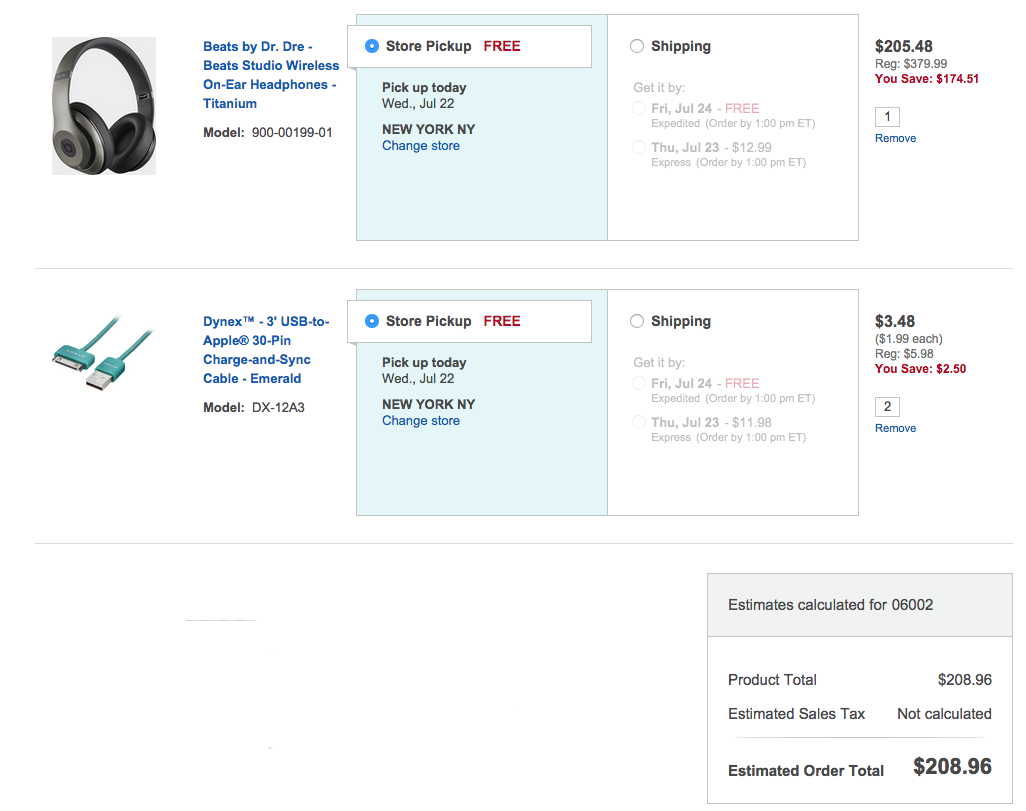The image, sourced from a website, depicts a detailed breakdown of an online order for two computer-related items. The first item, displayed in a light blue section, is a pair of black Beats by Dr. Dre Studio Wireless On-Ear Headphones in Titanium. The model number is specified, and the pickup option is highlighted as "store pickup" with an availability of "free pickup today," dated Wednesday, July 22nd, in New York, New York. There is an option to change the pickup location by clicking a designated area.

Adjacent to this, in a white section, there are shipping options outlined: standard free shipping by Friday, July 24th; expedited shipping by Thursday, July 23rd, for an additional $12.99; and an option for expedited shipping by Friday, July 24th if ordered by 1:00 PM ET. The listed price for the headphones is $205.48, with a quantity of one.

Below this, the second item is presented: the Dynex 3-Foot USB to Apple 30-Pin Charge and Sync Cable in emerald green. This item shows a store pickup option for $3.48 each, with a purchase quantity of two. The summarized total price for the order is $208.96. The visual elements suggest a straightforward and user-friendly interface for reviewing and modifying purchase details and shipping/pickup options.